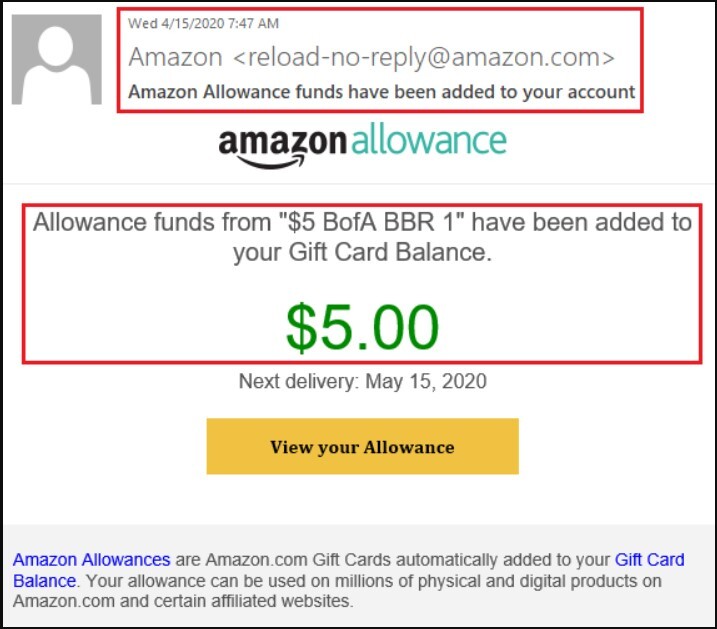Here is a detailed and cleaned-up caption for the image described:

---

The screenshot captures an email from Amazon, dated Wednesday, April 15, 2020, at 7:47 a.m. The sender's address is reload-no-reply@amazon.com. The email header reads "Amazon Allowance Funds have been added to your account" in black font, bordered by a red rectangle. Beneath this, the black Amazon logo is displayed next to the word "Allowance" in light blue font. The body of the email, in gray font, states: 'Allowance Funds from "5$ B of A, BBR1" have been added to your gift card balance.' Highlighted in the next section, large green text depicts the amount, "$5.00," also enclosed in a red rectangle. Below that, the text reads "Next Delivery May 15, 2020." An orange rectangle at the bottom with black font contains the call-to-action "View Your Allowance." The lower portion of the email includes a light gray border with "Amazon Allowances" in blue font, presumed to be a hyperlink. The message concludes with a note about the automatic addition of gift card balances and the availability of the allowance for millions of physical and digital products on Amazon and affiliated sites.

---